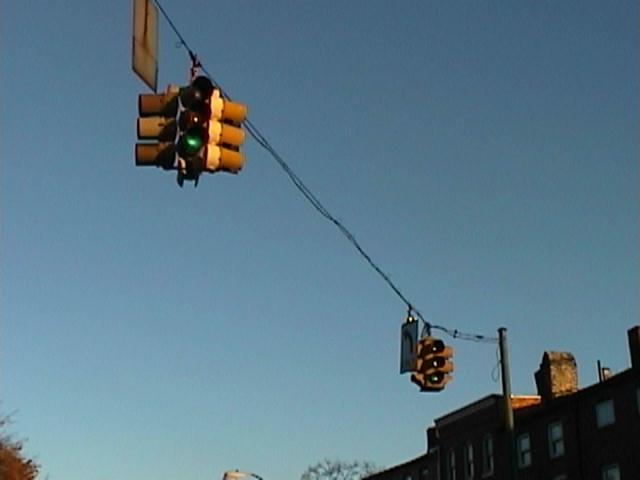The image depicts a traffic light suspended from a wire, with two signal lights prominently displayed. The traffic light closest to the viewer is glowing green, while the color of the more distant light is indiscernible. Both lights are attached to a horizontal pole and accompanied by hanging signs. The sign nearest to the viewer shows only its rusted back, whereas the farther sign features a left-pointing arrow. The scene is set beneath a blue sky with greenery visible—trees tower over a nearby, aged apartment building, which has its windows adorned with drawn blinds. Additionally, a tree occupies the lower left corner of the frame, adding a touch of nature to the urban landscape.